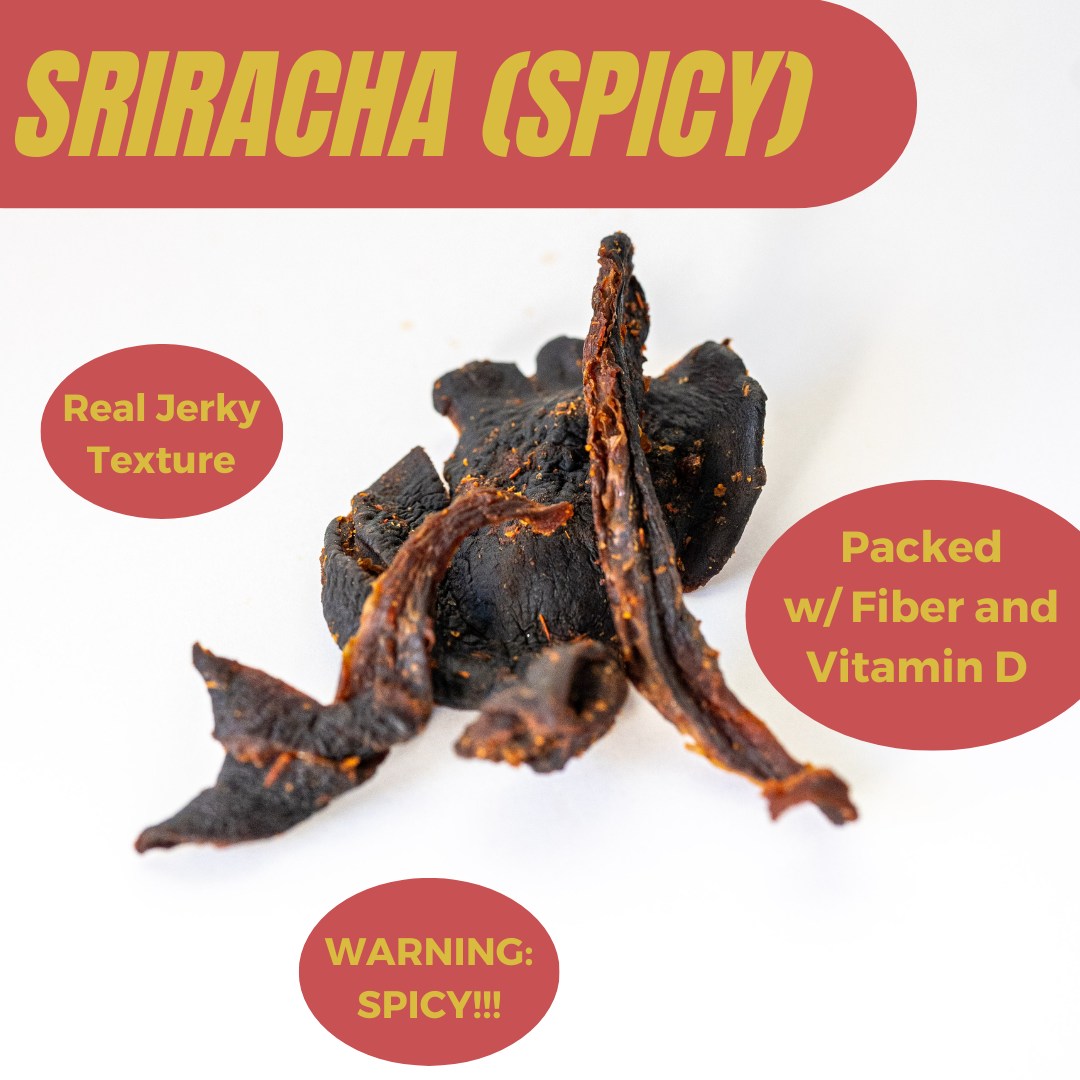The image is an advertisement for sriracha-flavored beef jerky set against a white background with a slight blue tinge at the top. At the upper left, within a red rectangle with a rounded end on the right, the word "SRIRACHA" is prominently displayed in yellow, followed by "(spicy)" in parentheses. Below this, on the left, is a red oval containing the text "Real jerky texture" in yellow. The center of the ad showcases several dark charcoal-colored beef jerky strips, with hints of brown, stacked in a pile. Some pieces lean against the mound, and the jerky appears dried with visible herbs and spices. To the right of the jerky, another red oval reads "Packed with fiber and vitamin D" in yellow. Beneath the jerky, a final red oval warns "Warning: spicy!!!" in yellow letters. The jerky is described as having a real jerky texture, packed with fiber and vitamin D, and is marketed for its spicy sriracha flavor.